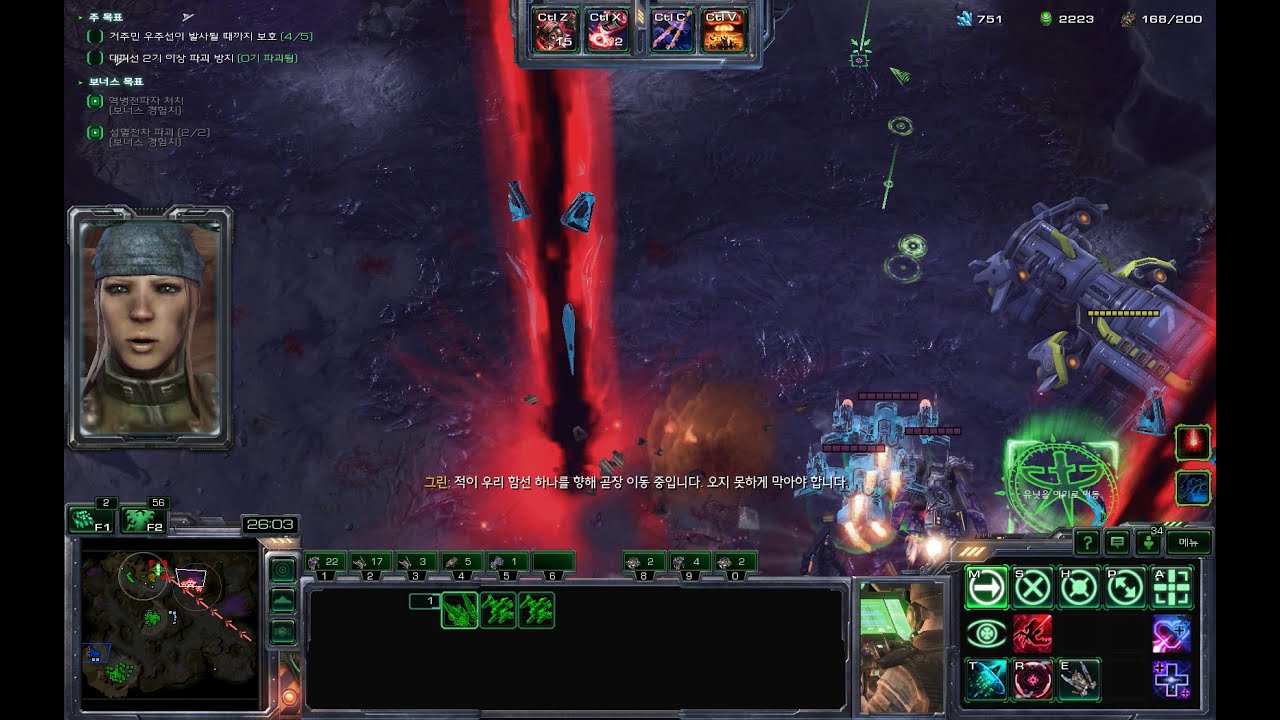The image is a detailed screenshot from the real-time strategy video game StarCraft 2, illustrating a richly informative heads-up display. At the bottom edge, there are multiple control panels: on the lower left, a small map showing battlefield overview; on the lower right, a menu with specific commands such as moving and attacking. The HUD features text that is likely in Chinese or Japanese and includes function keys, suggesting this game is played on a computer. On the left, there's an animated character's profile picture, which seems to represent either the player or an in-game character. The main visual depicts a top-down view of a dark blue, cave-like landscape with water droplets falling onto the surface. Dominating the scene is a striking red column of energy rising dramatically from the ground.